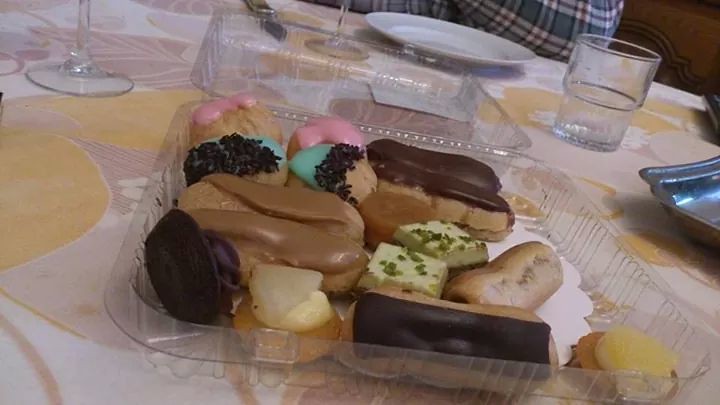This image depicts a colorful and inviting table setting, centered around a clear, square plastic container filled with an array of delectable desserts and pastries. The tabletop is adorned with a white tablecloth featuring various yellow circles in a playful pattern, intermingled with soft pastel hues of orange and pink. Positioned in the background is a regular-sized, empty white dinner plate. To the right side, a standard drinking glass can be observed, half-filled with water, and the bottom portions of two stemmed wine glasses are visible, though their tops are out of frame.

The main focus of the image is the open plastic container in the center. Inside, a variety of sweets are neatly arranged, including donuts with different frosting colors such as pink and chocolate, eclairs, and cream puffs adorned with white frosting and sprinkles. Additionally, there are small cupcakes, brownies with green frosting, and cookies covered in icing. Beside this container, there is another clear serving tray which is empty, and a silver tray is placed at the corner of the table, further contributing to the overall presentation. The desserts within the container are diverse, with mentions of flavors and colors that emphasize the assortment and the festive feel of the spread.